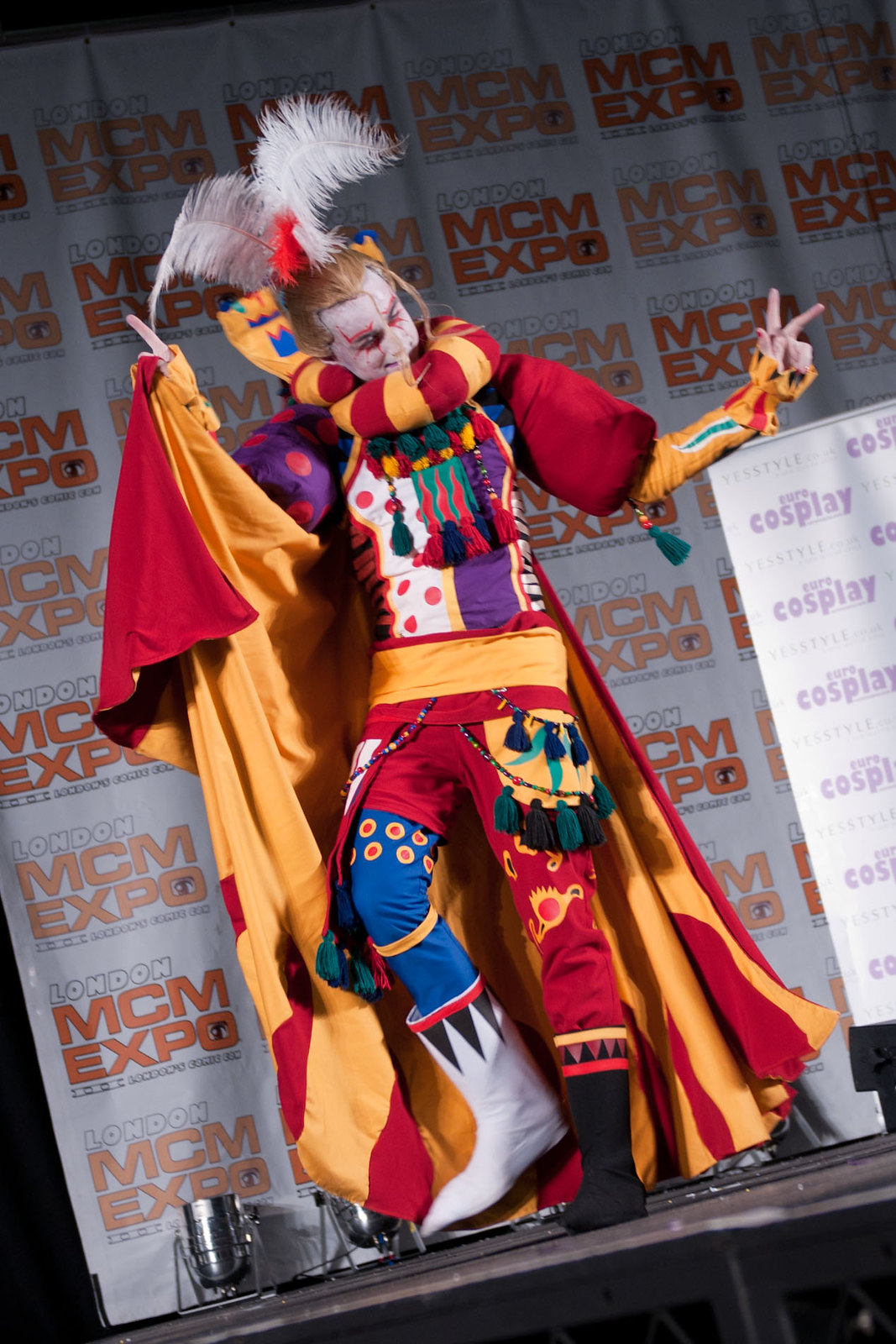A vibrant cosplayer stands on a black stage against a white backdrop repeating the text "London MCM Expo" in orange and off-white. Dressed in an eclectic jester-like costume, the performer commands attention with their striking face painted white and adorned with red accents above and below the eyes, reminiscent of Japanese Kabuki makeup. Blonde hair, topped with two white feathers and one red feather, adds to the whimsical appearance. The intricate outfit includes a multi-colored shirt featuring white, purple, and red circular designs, a heavy scarf with vertical red and yellow stripes around their neck, and an orange cape with red highlights. Their left arm points to the right, making a peace sign, clothed in red fabric on the upper arm and yellow on the lower arm. The ensemble also features an orange belt and pants split in color—one leg red and the other blue. The standout footwear consists of one white boot and one black boot. The vivid description is complemented by various tassels hanging from the neck, adding to the chaotic yet captivating look. Nearby, a piece of paper inscribed with "COSPLAY" in purple letters rests just beneath their hand.